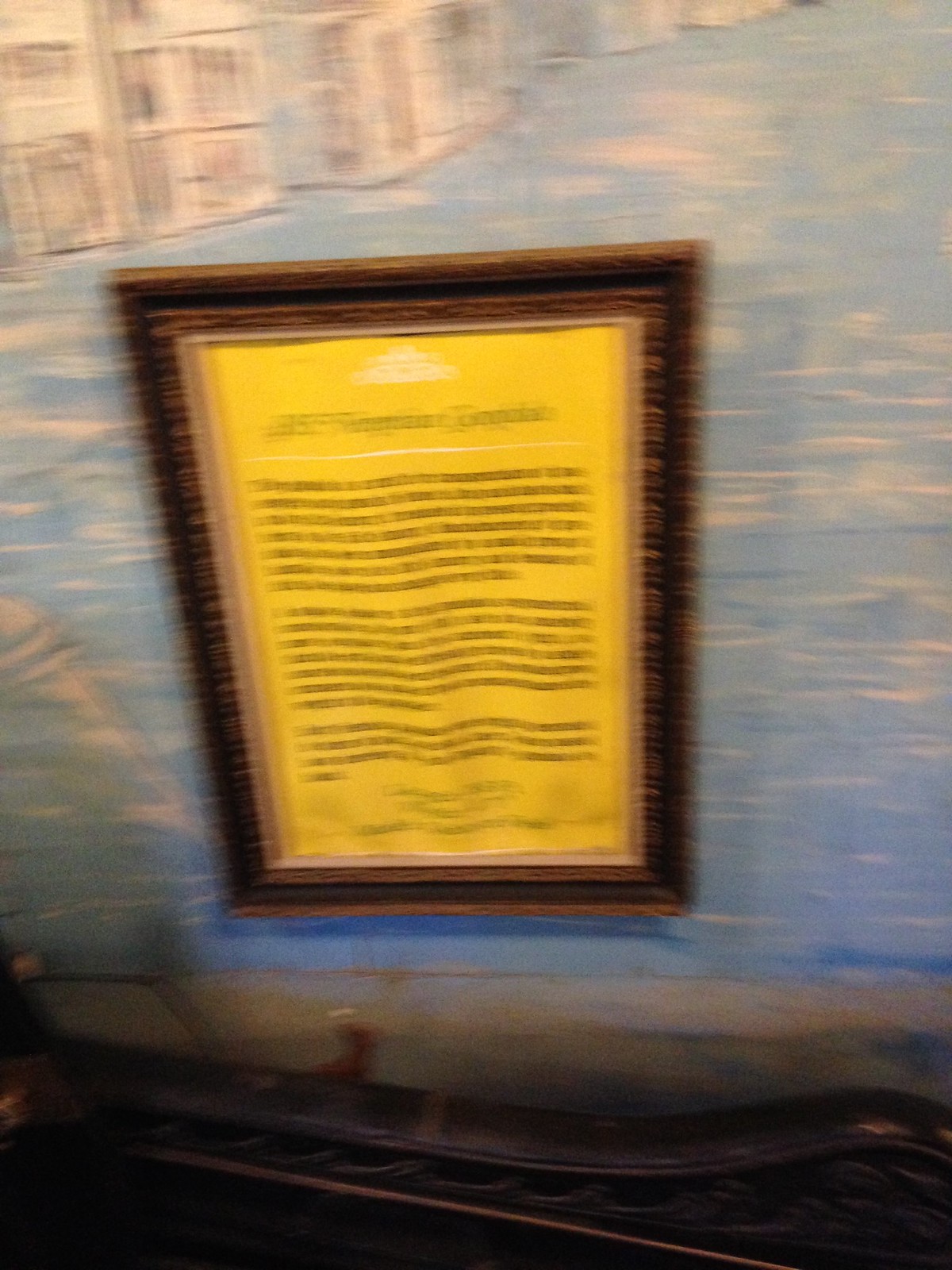This close-up image captures an intricate painting reminiscent of a Venetian scene. Despite the slight blur, the artwork vividly depicts a scenic street partially submerged in water, characteristic of Venice's unique charm. Prominently featured is a narrow canal with gondolas, specifically spotlighting a gondola in the lower section. The gondola bears a figure outlined in red, donning a distinctive white cap as he sits gracefully in the vessel. Centrally placed within the artwork is a framed document, though the text remains indistinct due to the blur. The document, rendered on yellow paper and encased in a rustic brown wooden frame, adds an intriguing historical element to the piece. The overall composition exudes a nostalgic aura, transporting viewers to the canals and waterways of Venice.